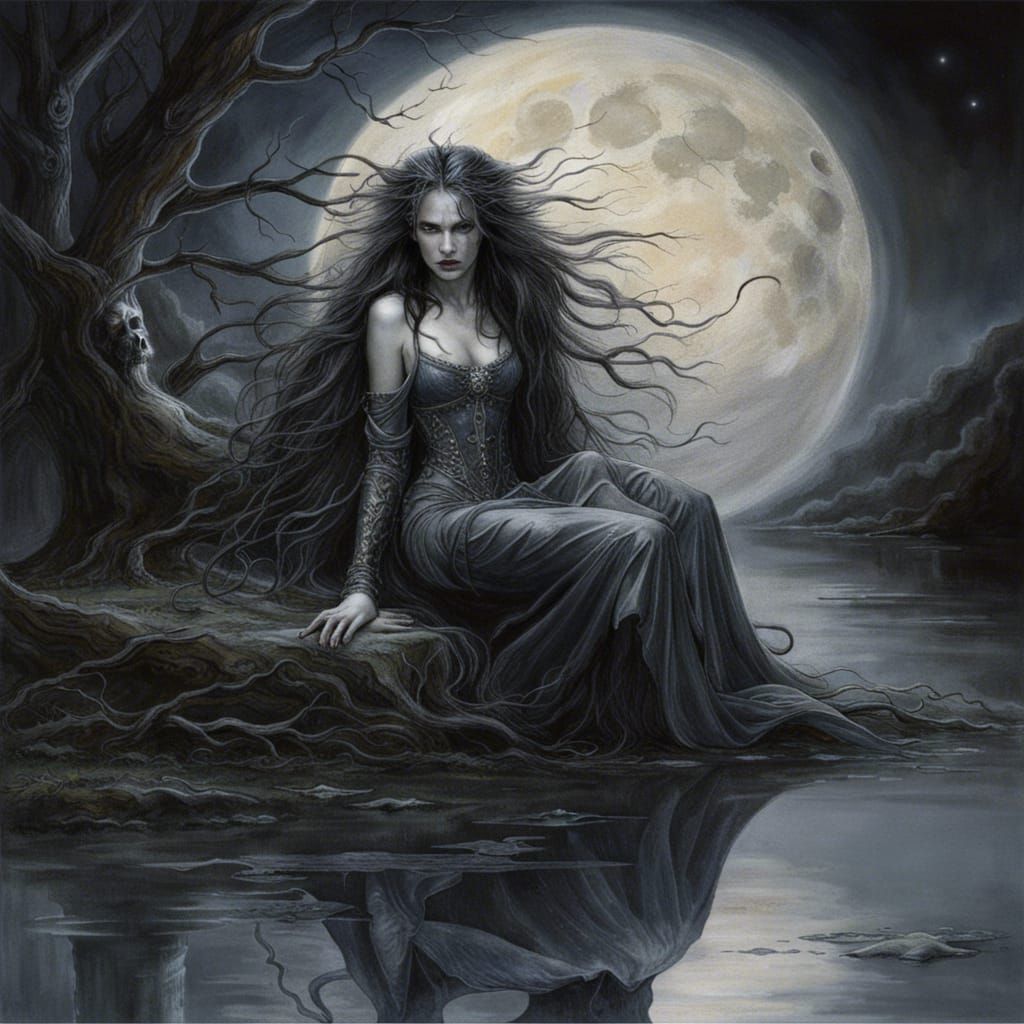The image is a square-shaped artistic representation, measuring approximately six inches by six inches, and embodies a haunting Gothic, fantasy aesthetic reminiscent of Dungeons & Dragons. Dominated by monochrome shades of gray, the scene portrays a ghostly, fiercely beautiful woman with an air of malevolence. Her extremely long, straggly black hair, resembling tree branches or electrified tendrils, flows wildly around her. Dressed in a strapless, form-fitting gown with corset detailing and off-the-shoulder sleeves, she sits perched on the edge of a gray, reflective swamp. Her feet nearly touch the inky water, casting a mirrored image back at her.

To her left, a gnarled, dead tree looms with a skull-like visage embedded within its trunk. The entire environment, from the trees to the water, is bathed in darkness, illuminated only by a dominatingly large, glowing yellow full moon that hangs prominently in the sky, casting an eerie light over the scene. This spectral moon is the sole source of color, contrasting starkly against the otherwise muted palette. The woman’s fierce expression enhances the image's haunting, ghost-like quality, adding an element of foreboding to the overall composition.